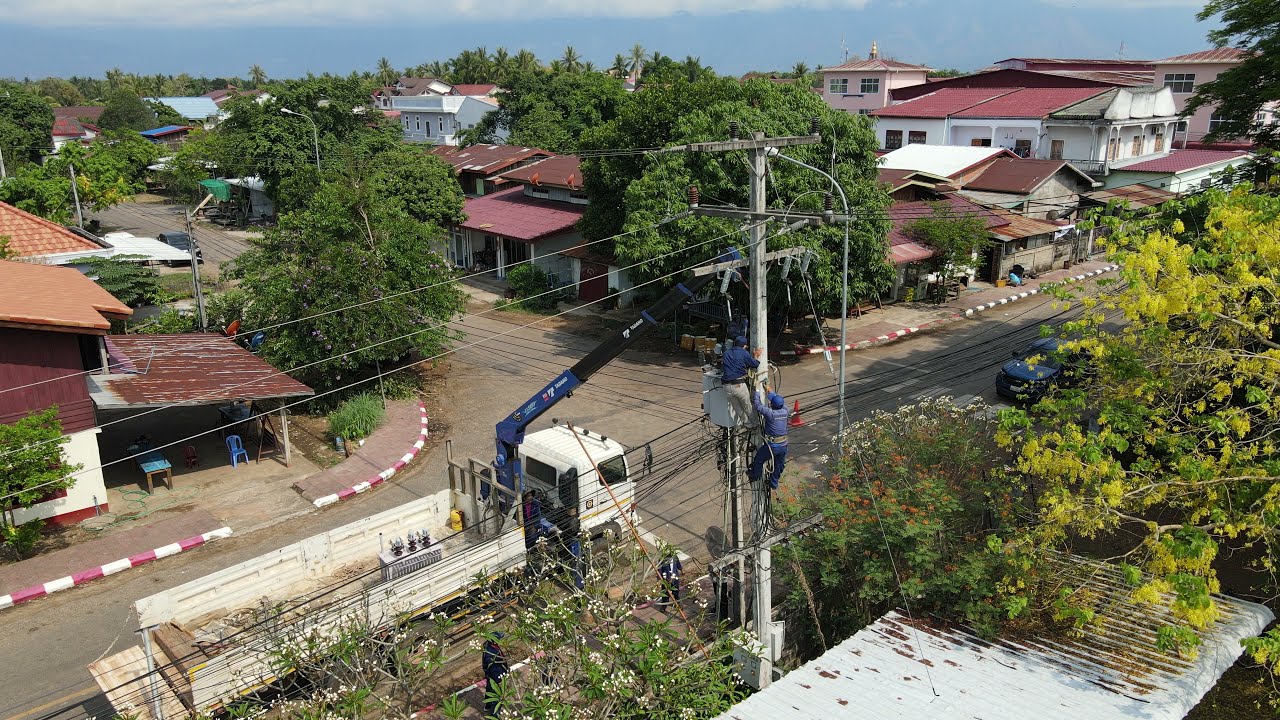Captured from a drone's perspective, this image showcases a bustling neighborhood with a distinct tropical ambiance. At the center, a white, elongated commercial truck is parked, featuring a blue crane arm that extends toward a central power line. Two workers, dressed in all blue, including their hats, are elevated by the crane; one is inside the bucket, while the other appears to be holding onto it. Surrounding the main scene, run-down buildings with red roofs and white walls populate the area. These structures vary from single to two-story residences and are complemented by scattered trees and clean yet rust-touched roads. The sky above is dotted with clouds, adding to the daytime setting. The overall palette includes hues of white, blue, green, red, orange, gray, and black, enhancing the vivid yet rustic quality of the neighborhood.